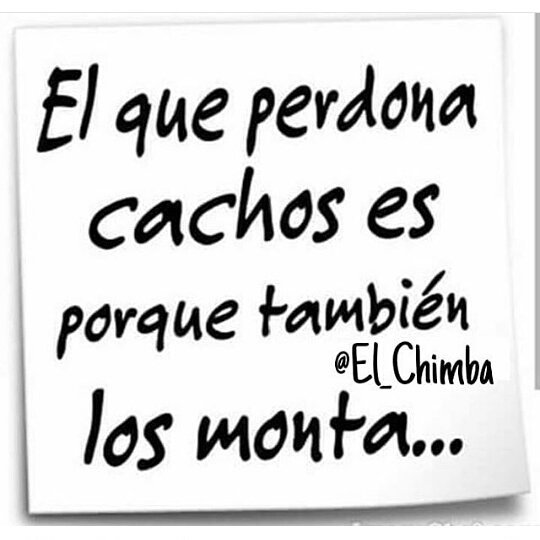This graphic resembles a digitally created post-it note with a slightly tilted, white square paper design, giving the illusion of the bottom right corner being lifted by using subtle gray shadow effects. The main text on the note is in large, black, handwritten-style font and reads: "El que perdona cachos es porque también los monta..." Above the last word of this phrase, cramped into the space, is the social media handle "@L_Chimba" in a less bold, uppercase black font. The entirety of the note maintains a simple and clean aesthetic with no additional elements on the white background, focusing solely on the Spanish saying and the handle.